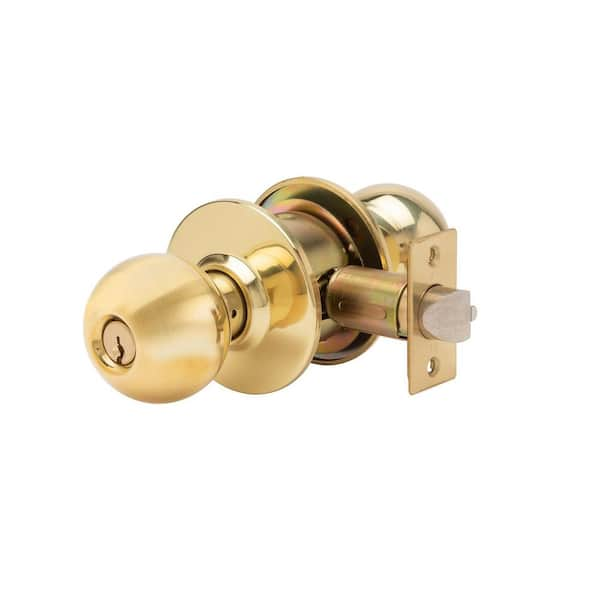This is a detailed photo of a complete bronze doorknob assembly, centered against a white, transparent background, reminiscent of what you'd typically find in a hardware store catalog like Lowe's or Home Depot. The image showcases both sides of the doorknob set, highlighting the shiny, light gold/bronze finish. On the left side of the image, you see the round doorknob with light reflecting off its surface, featuring a silver keyhole in its center. This keyhole is part of a more silver central cylinder. The assembly includes the gold-colored rounded area that attaches to the door. In the middle, you can observe the mechanism, including the latch that secures the door and extends outward. On the right side, the assembly mirrors the left with another doorknob and the locking mechanism. The entire setup is detailed, showing the bolt and all components necessary for installation, though there are no labels or brand indications on the image.